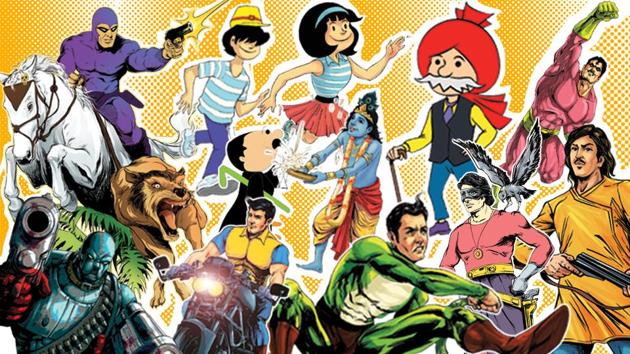The image is a vibrant, poster-style art design featuring a diverse assembly of cartoon characters and superheroes, all outlined in white against a yellow backdrop with a crisscross pattern of darker yellow gold. On the far left, riding on a white horse, is The Phantom, dressed in his signature purple suit and holding a gun in his left hand while gripping the rein with his right. Below him, a blue, metal-like bald man with red gloves and a bandolier of bullets across his chest wields a large gun, flanked by a growling wolf. To the right, a man in a yellow collared shirt with blue short sleeves rides a motorcycle. Next to him stands a man in a green bodysuit with brown boots and undershorts. Another notable character in the middle is a man with black hair and a black mask, in a red long-sleeve shirt, gold medallion, gold belt, and purple pants, with a black bird on his shoulder. 

In the upper section, a boy and a girl in white and blue striped shirts are depicted, with the boy wearing a yellow cap and the girl in a red skirt with a blue bandana. Below them is an Indian deity-like figure with blue skin, reminiscent of the Hindu god Shiva. Another figure, an older man with a white mustache and a turban, walks with a cane. In the upper right, a muscular man with black hair styled in a curlicue, a mustache, a pink uniform, green gauntlet gloves, and a green waistband hovers in the air, resembling superheroes from comic books like Shazam.

Lastly, at the lower right, there's an angry character holding a gun, adding to the diverse ensemble. Together, these figures create a dynamic and detailed collage of animated icons and superheroes from various genres and eras.